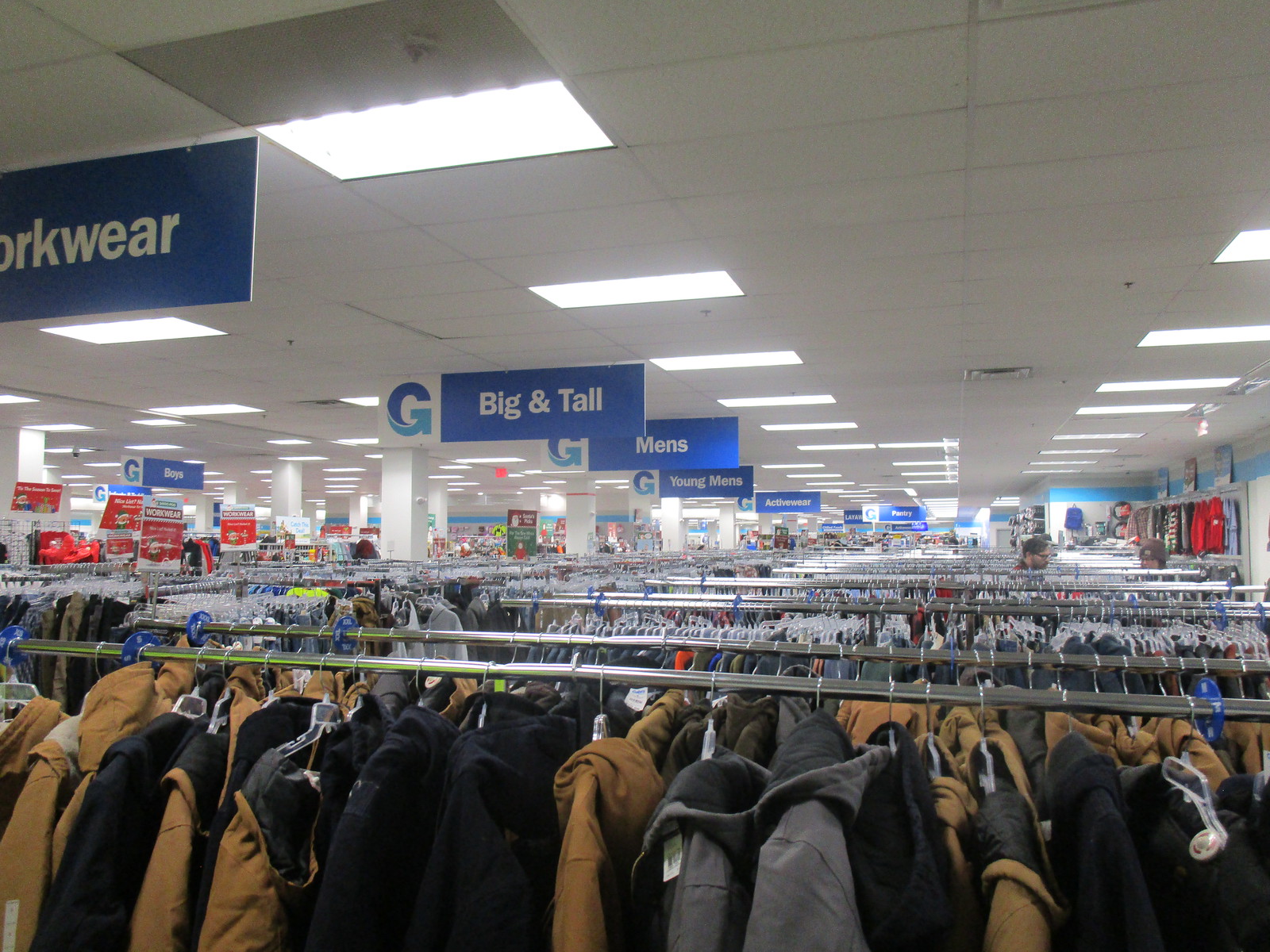This photograph captures the interior of a department store, offering a medium top view of rows of clothing racks that intensify in perspective toward the background. The store is illuminated by a dropped tile ceiling dotted with rectangular fluorescent lights arranged horizontally in line with the tiles. Prominent blue and white rectangular signs hang from the ceiling, guiding shoppers to "work wear," "big and tall," "men's," "young men's," and "active wear" sections. The racks themselves are constructed from silver tubular metal. The rack closest to the camera features an assortment of jackets, including black, brown, and gray Carhartt-style coats. Beyond that, another row displays hoodies in various shades such as black, brown, blue, and red. Off to the far right, red signs and white-painted support columns are visible, adding to the structured layout of the store. The sign "boys" can also be seen in the distance, indicating another section of the store.